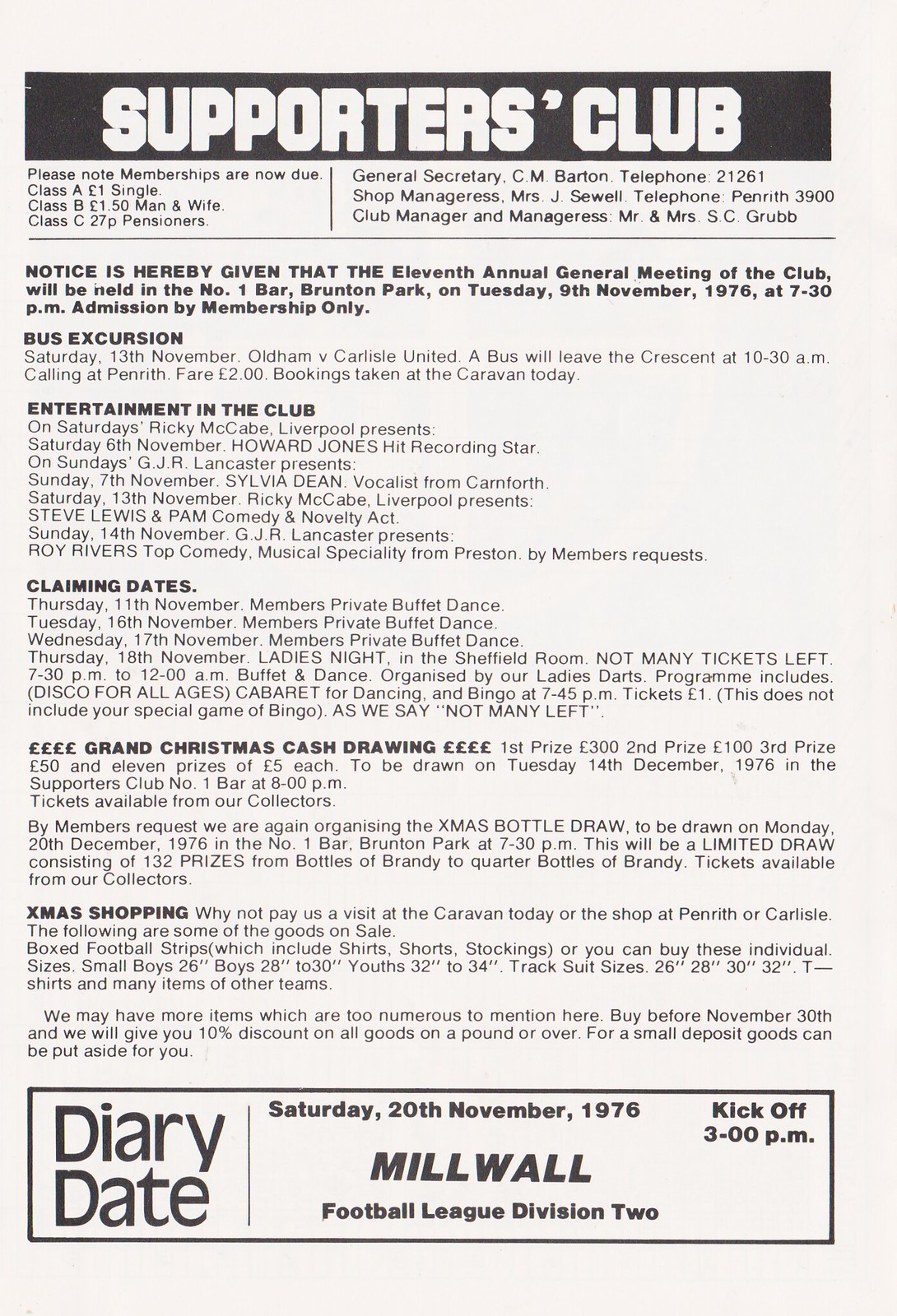This black-and-white image features a page from a game day program or magazine primarily promoting a club event. Dominating the top of the page, a bold black bar with large white text reads "Supporters Club". Beneath this, detailed in small text, is important business information listing roles such as the general secretary, shop manager, club manager, among others, along with various types of memberships and dues.

The central portion of the page is packed with several blocks of text. It starts with a prominent announcement in bold: "Notice is hereby given that the 11th annual general meeting of the club will be held in the Number One Bar, Brunton Park on Tuesday, 9th November, 1976 at 7.30pm, admission by membership only." This is followed by essential details regarding a bus excursion, entertainment in the club, upcoming claiming dates, a grand Christmas cash drawing, and Xmas shopping.

At the bottom of the page, encapsulated within a thin black-lined box, "Diary Date" is displayed in bold black text on the left. To the right, specific event information is listed, noting a Saturday fixture on 20th November, 1976, with a kickoff at 3pm for a Millwall Football League Division 2 match.